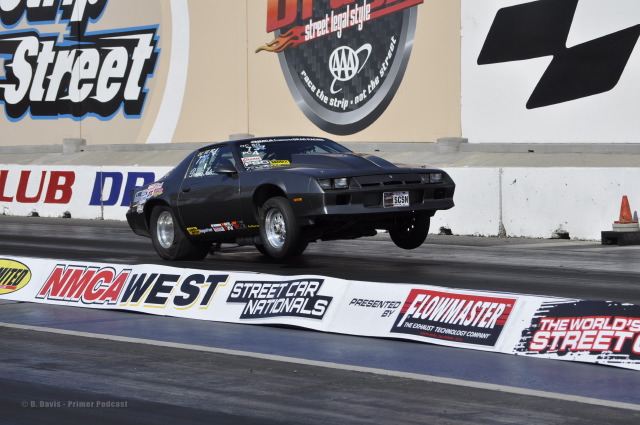The image captures a deep blue muscle car racing on a drag strip, its front wheels airborne, emphasizing the car's high speed and power. The car, likely in a left-front profile, is adorned with various small decals, including those on the passenger side door, upper right windshield, and left rear fender. The racetrack is bordered by a series of white advertising banners. Prominent logos include NMCA West, Street Car Nationals presented by Flowmaster, and phrases like "The World's Street" and "Street Legal Style." The backdrop features a tall, beige wall with additional logos, some partially obscured. The car's license plate reads SC5N, further personalizing this high-octane scene. The vivid detail from three perspectives combines to provide a unified, dynamic snapshot of the racetrack environment.